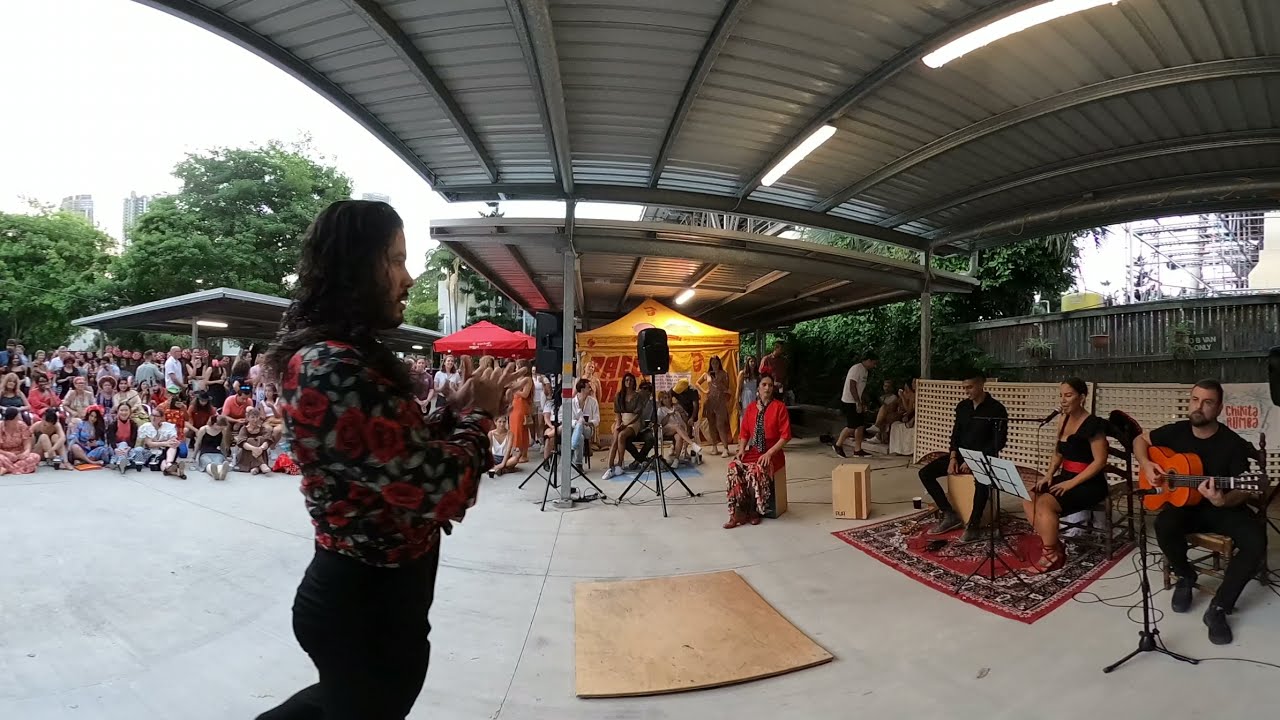The photograph captures an outdoor musical performance under a metal awning. On the right side of the image, a small band of four individuals is seated on wooden crates atop a red carpet. The band consists of a guitarist with an orange/red acoustic guitar dressed in black, a Latina woman vocalist in a black dress with a red belt singing into a microphone, a bongo player also in black, and another man in black clothing who appears to be simply enjoying the music. At the front, standing and clapping, is a man with long curly black hair wearing a fancy floral rose-patterned shirt in pink and red hues with black pants. The audience, a mix of seated and standing people, is visible on the left side of the photograph. They watch the performance attentively from under red and yellow tents, with a backdrop of trees and distant buildings. A black speaker box is placed centrally in the viewed scene.